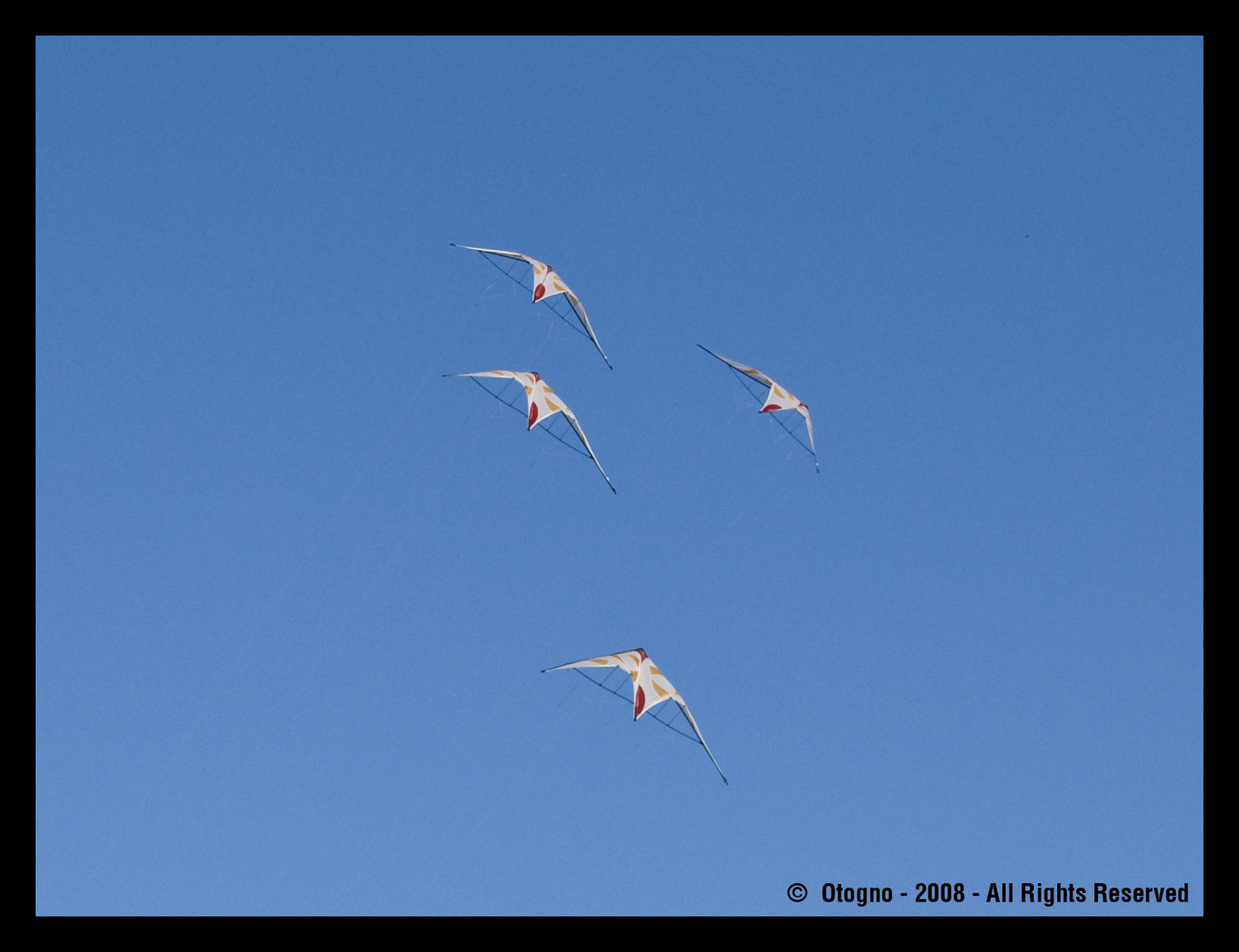The image features a clear blue sky devoid of clouds, showcasing four professionally flown kites. The kites, which are about three feet in size and shaped like birds with wings spread out resembling seagulls, are predominantly white with distinct orange and red triangular patterns, and black structural piping. These kites are soaring gracefully, mostly in the same direction, except for one veering slightly to the right. The sky scene is framed by a black border, and at the bottom right corner, there's a copyright notice in black lettering: "© O-TOGNO-2008-All Rights Reserved", with specific capitalization on the 'A', 'R', and 'O' as noted. Two kites are positioned closer together near the upper left corner of the image, while the other two are more spaced out near the lower right corner.